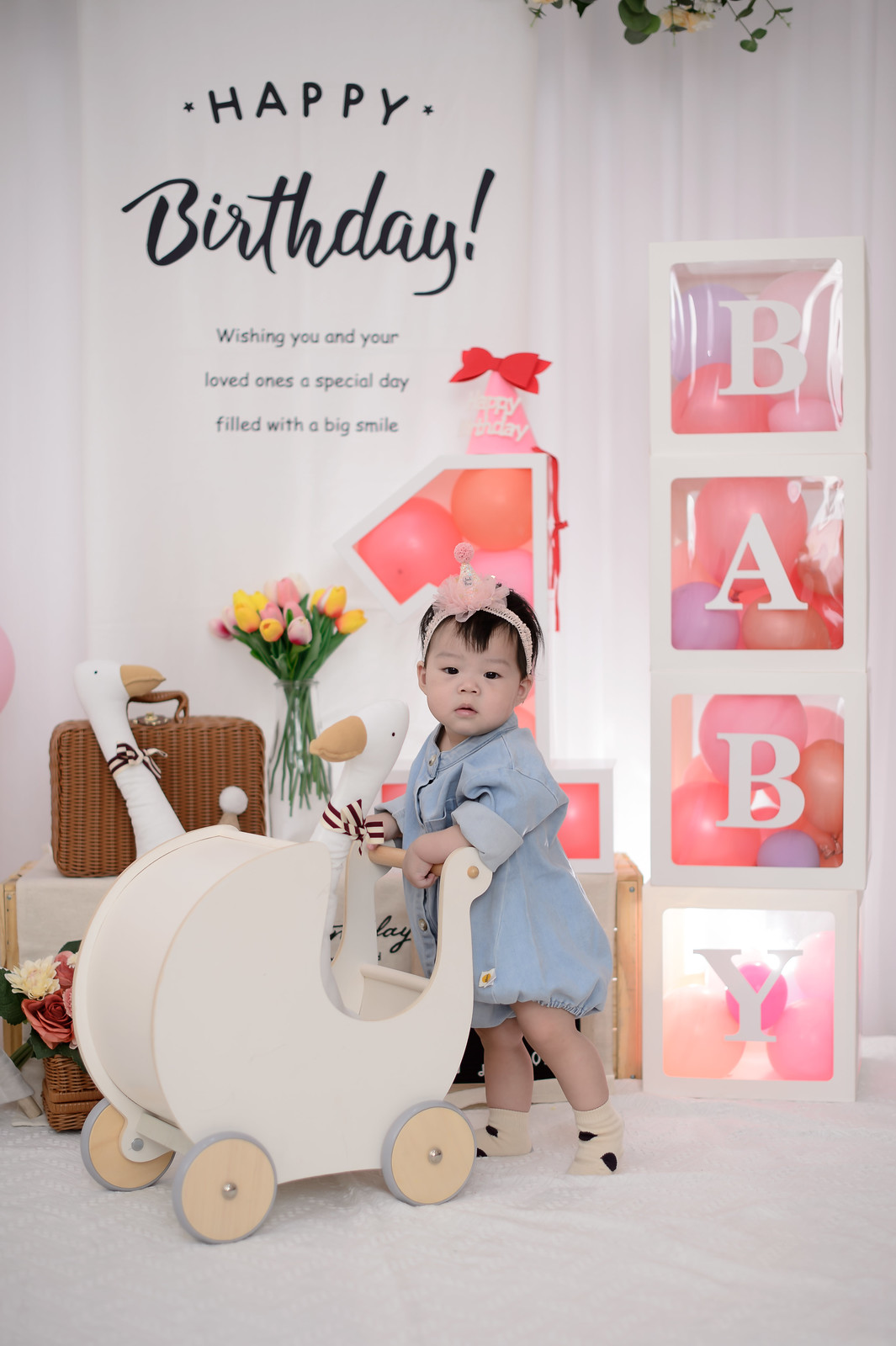In this professionally posed and well-lit photographic image used as a happy birthday card, a delightful scene captures a young Asian girl, approximately two years old, radiating joy. She is dressed in an adorable blue denim baby dress paired with black and white socks and a cute pink headband. Enthusiastically, she pushes a white baby carriage with wooden wheels that features two stuffed geese inside. 

To her right, stacked clear blocks spell out "BABY," each block filled with colorful balloons. Behind her is an elegantly arranged table adorned with a wicker suitcase, a stuffed goose head, a vase of tulips in various colors (yellow, pink, and white), and a towering cluster of balloons capped with a birthday hat that reads "HAPPY BIRTHDAY." The setting is a cozy, likely a baby's room, with pristine white walls and a lush white carpet underfoot.

Prominently displayed at the top of the card is the cheerful message: "HAPPY BIRTHDAY, wishing you and your loved ones a special day filled with a big smile." This image beautifully combines the celebration's joyful spirit with the innocence of childhood, making it a perfect birthday greeting.